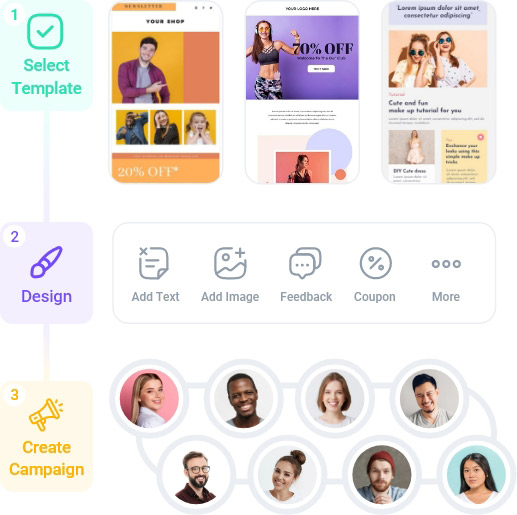The image appears to be a detailed screenshot of a webpage with multiple elements, likely related to creating marketing campaigns or templates:

1. **Overall Page Layout:**
   - **Background:** White.
   - **Zoom Level:** 150% for better clarity of the details.
   
2. **Top Section:**
   - **Top Left Corner:** Features a square checkbox outlined in green with a green checkmark, labeled "Select template."
   - **Templates Display:** 
     - **First Template (Left):** An orange and yellow design featuring a young man with three smaller pictures of people underneath and a tag indicating "20% off."
     - **Second Template (Middle):** A young woman with long light brown hair, wearing a crop top, against a purple backdrop. This template shows "70% off" beside the image along with a circular picture of another woman below.
     - **Third Template (Right):** Two women with light skin and long hair wearing sunglasses, with an additional picture of a woman to the left underneath. A yellow rectangle appears to the right of this picture.
   
3. **Middle Section:**
   - **Step 2 - Design:** 
     - **Details:** Purple section indicated by a number 2 and an image of a paintbrush.
     - **Elements:** A central rectangle with grey icons representing various actions – "Add text," "Add image," "Feedback," "Coupon," and more.
   
4. **Bottom Section:**
   - **Step 3 - Create Campaign:**
     - **Details:** Written in yellow and indicated by a number 3 accompanied by a loudspeaker icon.
     - **Visuals:** Features eight connected circles outlined in grey, showcasing diverse individuals:
       - **Top Row:** 
         - Woman with light skin and blonde hair.
         - Black man.
         - Woman with light skin and dark hair.
         - Man with lighter skin, dark hair, and a beard.
       - **Bottom Row:** 
         - Man with lighter skin, glasses, and a beard.
         - Woman with light skin and a bun on her head, with dark hair.
         - Man with light skin, wearing a red cap, and a reddish beard.
         - Asian-looking woman with long dark hair, against a blue background.

This caption provides a comprehensive description of the screenshot, detailing the layout, colors, and individual elements present in the image.